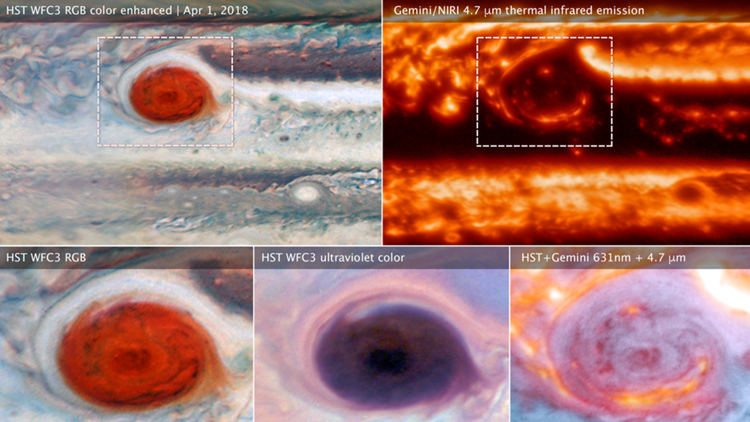The image is a composite array of five photographs capturing Jupiter's iconic Great Red Spot from different observational perspectives and wavelengths. The photographs are organized into two rows, with the upper row containing two images and the bottom row containing three. Each photograph features a white textual overlay on a gray translucent strip at the top:

1. The top-left image, labeled "HST WFC3 RGB color enhanced, April 1st, 2018," presents a vivid color-enhanced view of Jupiter's red storm, bracketed by a dashed rectangle. "HST" likely denotes the Hubble Space Telescope.
2. The top-right image is a "Gemini NIRI 4.7 thermal infrared emission" capture, showcasing a swirling pattern of blue, white, and purple with the red storm prominently highlighted. It appears to originate from the Gemini observatory.
3. The bottom-left image mirrors the upper left but zooms in on the storm itself, also marked as "HST WFC3 RGB."
4. The bottom-center photograph is taken using ultraviolet sensors, labeled "HST WFC3 ultraviolet color." Here, the storm is depicted in deep blue shades with pink surrounding clouds, diverging from the usual red appearance.
5. The bottom-right image combines data from both Hubble and Gemini, noted as "HST Gemini 631NM plus 4.7 UM." This image presents the storm with pink and orange hues, resembling the thermal characteristics seen in the upper-right image.

Together, these images offer a comprehensive, multi-spectral view of Jupiter's Great Red Spot, highlighting its dynamic features across various wavelengths and observational techniques.